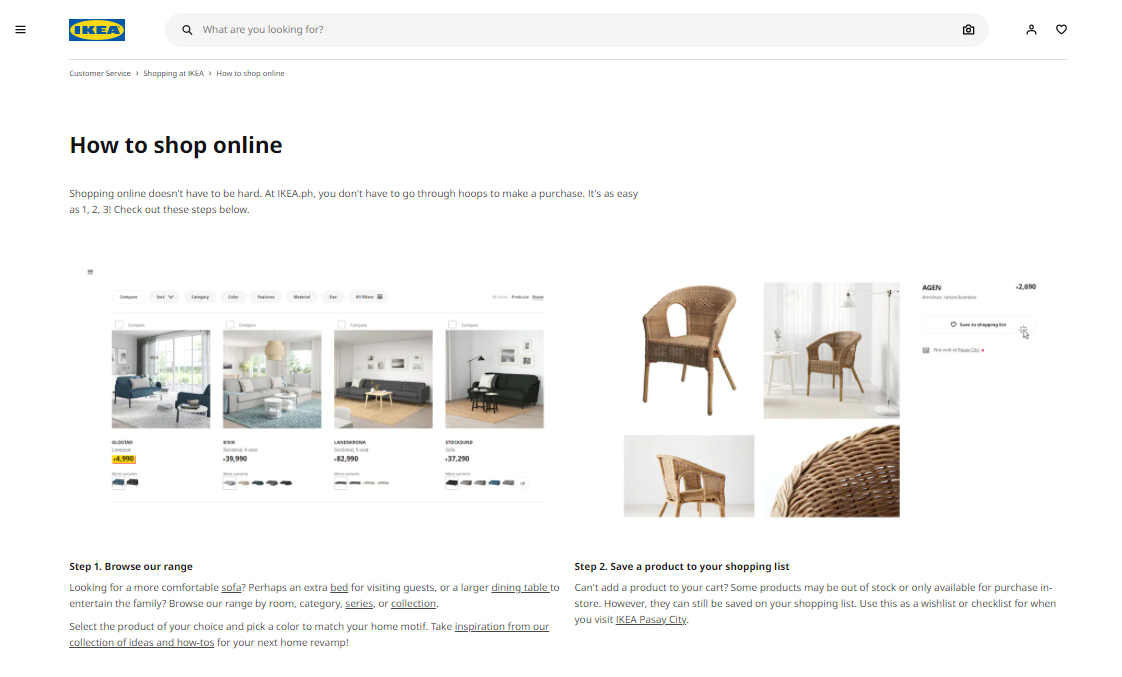**Detailed Caption for IKEA Online Shopping Guide Image:**

The image captures the sleek and user-friendly IKEA website interface, dedicated to guiding customers through their online shopping experience. The webpage prominently displays the helpful title, "How to Shop Online," aimed at assisting those new to digital shopping platforms. It reassures users that purchasing from IKEA online is straightforward and hassle-free. 

The main section of the website features vibrant, high-quality photographs of various rooms furnished with IKEA products. Key items showcased include two elegant black couches, a cozy living room setup with a chair and a couch, and another inviting space with a pristine white couch. Notably, the price tags are clearly displayed beneath each product, with one price highlighted in yellow, possibly indicating a sale or special offer.

The guide breaks down the shopping process into clear, easy steps:

1. **Step One: Browse Our Range** - Users are invited to explore IKEA’s extensive catalog, whether they seek a more comfortable sofa, an additional bed for guests, or a larger dining table for family gatherings. The platform allows customers to choose products in various colors to best match their home decor, encouraging inspiration from IKEA’s collection of ideas and how-tos.

2. **Step Two: Save Your Product** - After selecting a product, customers can easily add it to their shopping list or cart, streamlining the purchasing process.

The design of the website is commendably clean and uncluttered, enhancing the overall user experience. On the right side of the page, a featured chair is displayed from multiple angles, including close-up views. This allows potential buyers to scrutinize the material and construction quality, ensuring a well-informed purchase decision. 

Overall, the IKEA online shopping interface stands out for its clarity, simplicity, and detailed product presentations, catering to both novice and experienced online shoppers.